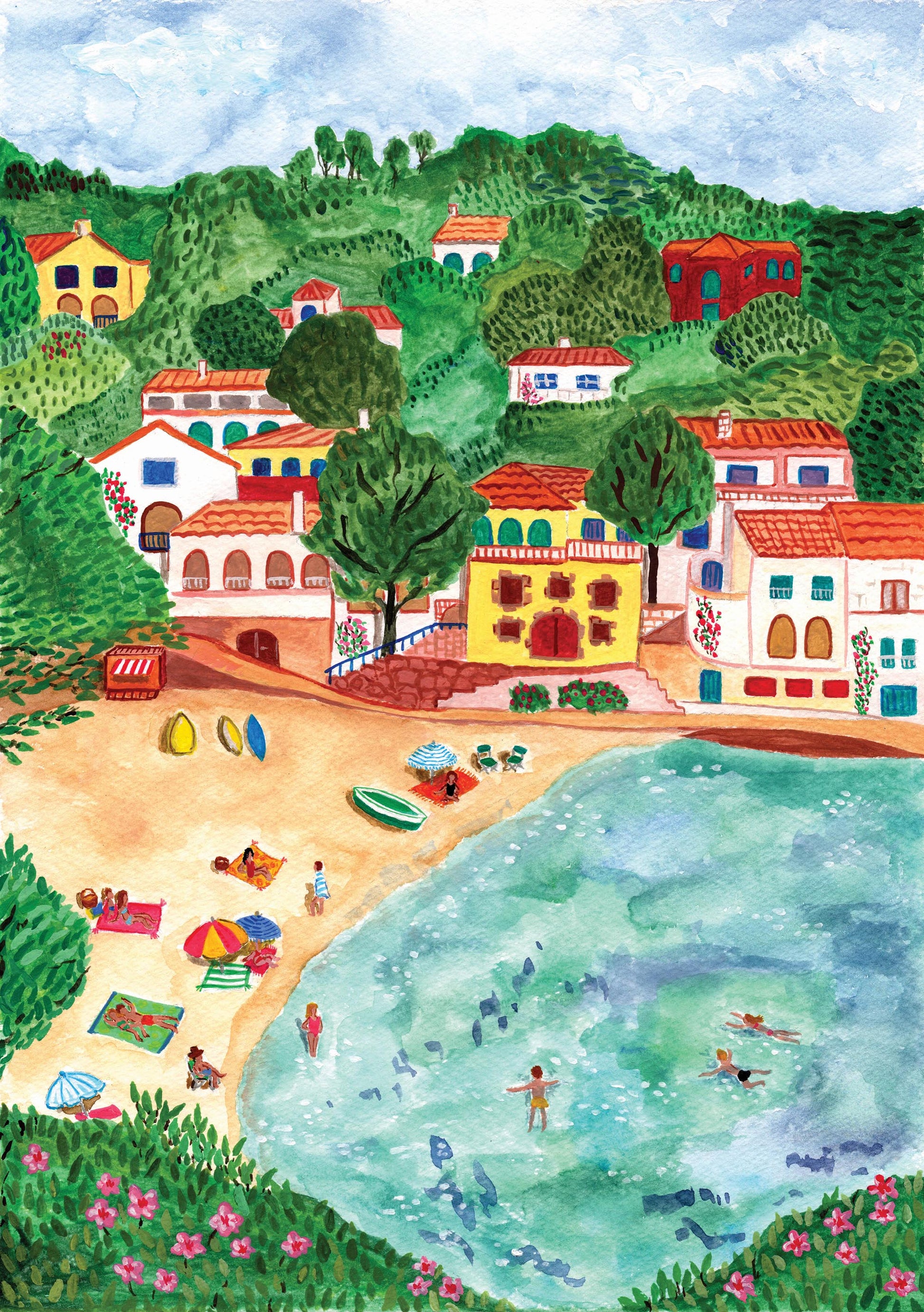This vibrant and colorful painting, possibly a watercolor, captures a picturesque beach scene set against a lush green hillside dotted with quaint, brightly-colored homes reminiscent of Spanish or Italian architecture. The houses, predominantly yellow, coral, and red with colorful windows and red roofs, are nestled among lots of greenery, including trees and flowering plants. In the foreground, a serene green and blue body of water, possibly part of the ocean, is flanked by a sandy beach where people are laying out on towels with umbrellas and surfboards or swimming in the water. The beach also features boats and beach blankets. Above the hillside, a clear blue sky with clouds completes this cheerful and lively scene, accented by vibrant yellows, pinks, blues, and purples, giving the image a distinctly bright and vivid appearance.